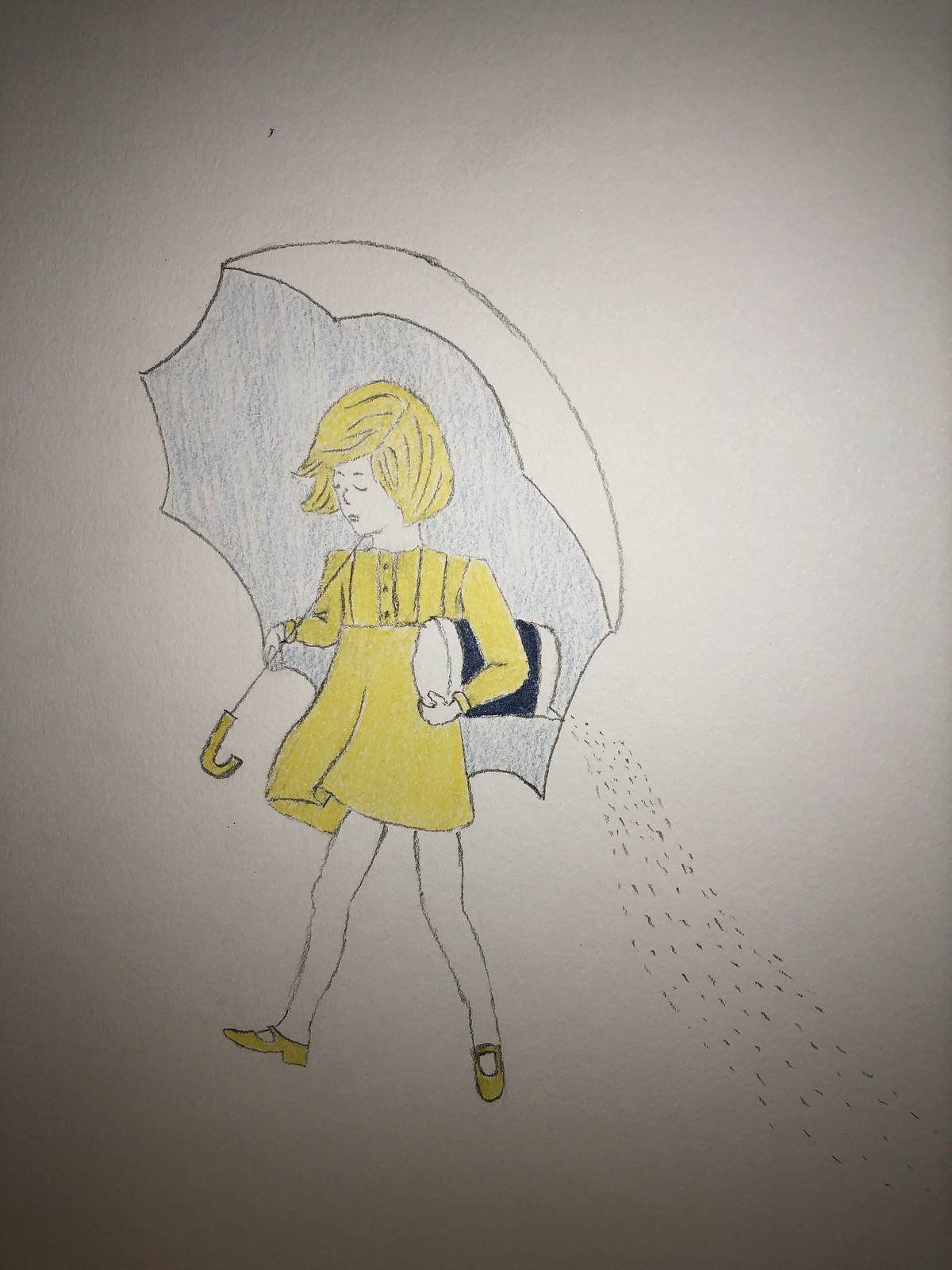The image is a detailed colored pencil drawing on a white piece of paper, possibly with some parts shaded due to printing issues. It depicts a young girl, who appears to be around ten years old, with blonde, short hair, and white skin. She’s wearing a bright yellow, short dress, accented with three buttons down the front and a couple of stripes, and yellow strapped sandals. The girl holds a large umbrella in her left hand; the umbrella has a white handle and a canopy that’s white on top with a light blue underside. A look of melancholy is evident on her face, characterized by closed eyes, a small nose, a small mouth, and two eyebrows, as she gazes downward. In her right arm, she clutches an oval-shaped container, blue in the middle and white at each end, resembling a Morton Salt container. The container tilts, spilling seed-like particles, possibly salt, behind her.